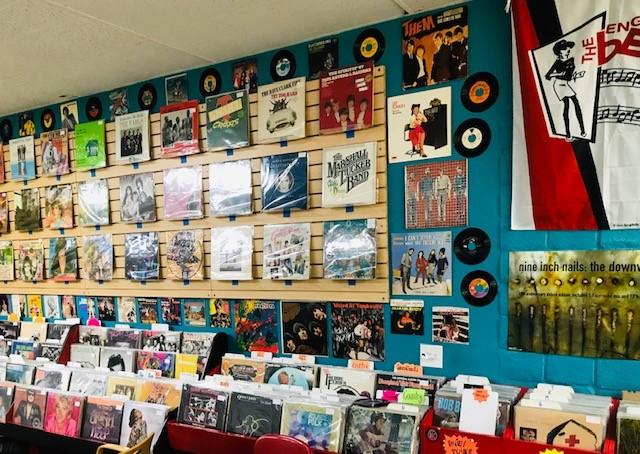The image portrays a vibrant, vintage record store with a turquoise blue wall adorned with an array of both full-size albums and 45 RPM records arranged in aesthetically pleasing patterns. The wall features approximately 15-20 albums displayed in neat lines, interspersed with decorative 45s that create an eye-catching design. Further into the store, a board displays additional albums, though their titles are indistinguishable due to distance. Below the board are categorized bins brimming with records, each separated by inserts for easy browsing. Among the decor, a striking poster catches the eye, depicting a girl in a white skirt, black tights, and a top, likely a go-go dancer, posed against a red and white flag backdrop. The store also includes notable posters like those for Nine Channels, Steve Miller Band, and the Marshall Tucker Band, juxtaposed against red shelves and a white ceiling, creating a nostalgic and lively atmosphere.